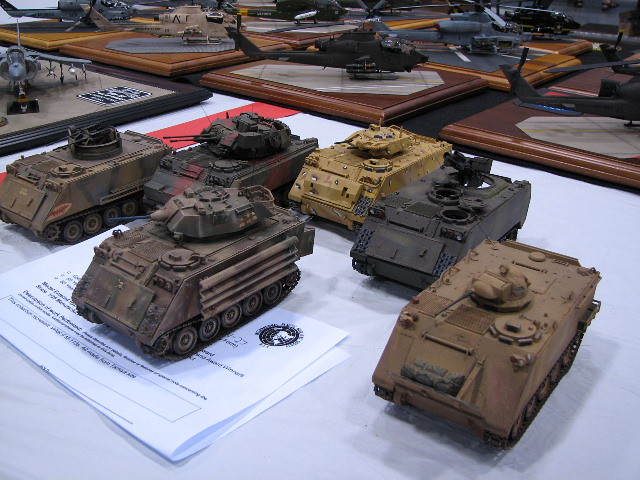This color photograph depicts a detailed display of various military toy figurines arranged on what appears to be a white display board or table. The focal point is six tank models, distinctly colored in muddy brown, charcoal gray, yellowish-puce, and army camouflage shades. These tanks are positioned in the middle, with a folded white piece of paper featuring tight print placed underneath one of them. Surrounding the tanks are multiple raised square bases, resembling plaques, each topped with different military aircraft figurines, including helicopters and airplanes in colors such as gray, black, beige, and a combination of black and white. In the forefront stands a white surface with a red strip, while behind it are brown outlined squares with gray centers, adding structure to the display.